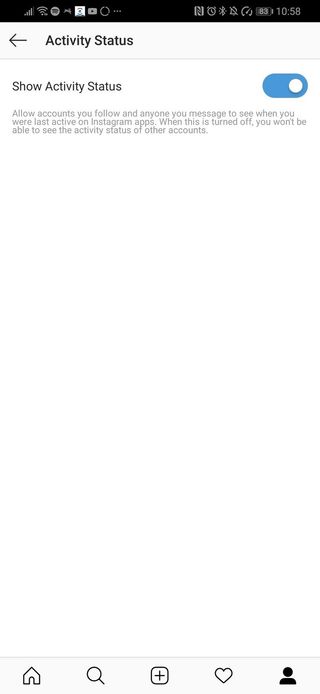This image is a screenshot from a tablet or smartphone, primarily depicting a settings screen for Instagram. 

At the top of the screen is a dark black bezel containing various status icons. On the left-hand side, these icons include:

- A signal strength indicator showing 3 out of 4 bars.
- A full Wi-Fi symbol.
- A circle with dark grey text.
- An unrecognizable white square with blue and black accents.
- A dark grey YouTube symbol featuring a black right-pointing arrow.
- A dark grey circle followed by three horizontal dots.

On the right-hand side of the bezel, the icons include:

- Two light grey "L" shapes pressed closely together.
- An alarm clock symbol.
- A Bluetooth symbol with a muted bell overlay.
- A grey speedometer.
- A battery icon displaying 83% in white.
- The time, shown as "1058" without AM or PM indication, suggesting military time.

Below the bezel, the main content of the screenshot shows a settings page related to Instagram's activity status. A mid-grey rectangle features a back arrow on the left, indicating navigation options.

The text within the settings page reads:

- "Show activity status" with a blue slider to the right, indicating the feature is turned on.
- In smaller grey text below, it explains: "Allow accounts you follow and anyone you message to see when you were last active on Instagram apps. When this is turned on, you won't be able to see the activity status of other accounts."

At the bottom of the screen, on the bottom bezel, there are various navigation icons for Instagram:

- A house symbol representing the home screen.
- A magnifying glass symbol for search.
- A square with a plus sign for adding new posts.
- A heart symbol for activity and likes.
- An icon of a person, consisting of a circle and an overturned half-circle, representing the user profile. 

The overall setting and details suggest that this screen is meant for adjusting and understanding activity status visibility within Instagram.